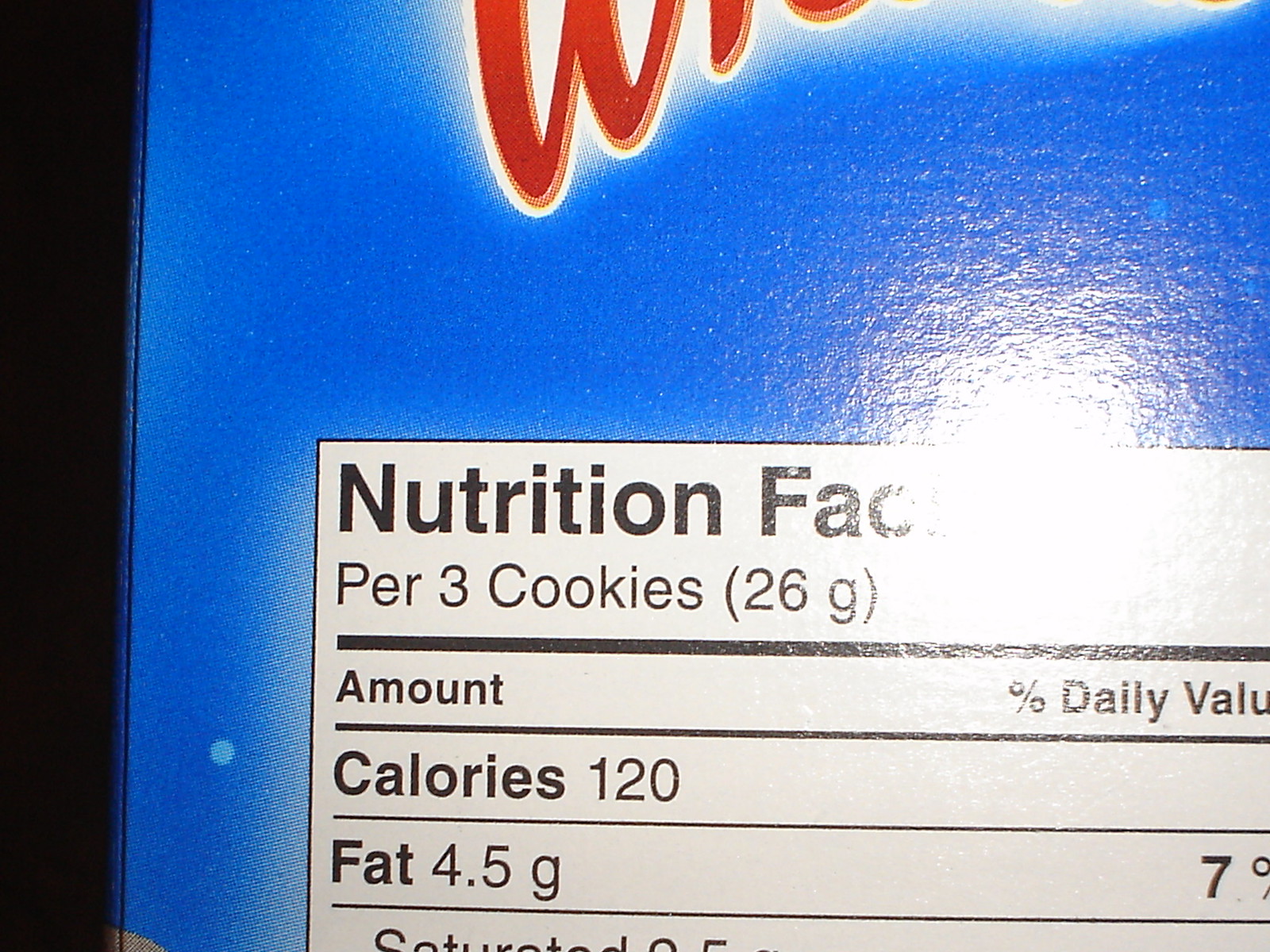Close-up photograph capturing a section of the Nutrition Facts label on an unidentified food package. The image is tightly cropped, revealing minimal brand information aside from a partially visible red "W" at the top center. The label is set against a blue background, with a camera flash creating a glare that partly obscures the text.

The visible Nutrition Facts include details for a serving size of three cookies (26 grams), stating the following information: Calories - 120, Total Fat - 4.5 grams (7% Daily Value). The word "saturated" is partially cut off, and there is a partial black strip along the left edge of the frame. The overall context is limited due to the tight crop and glare.